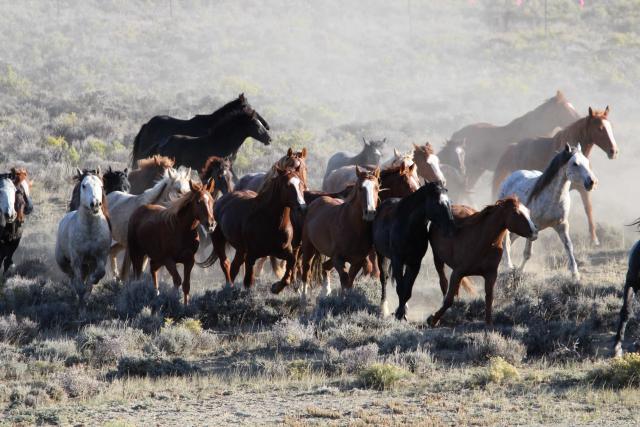This image depicts a photograph of a herd of wild mustang horses situated on a dusty plain with sparse vegetation composed of low green grasses and small plants. The majority of the horses are clustered towards the center of the image, creating a dynamic scene as they appear to be running or walking towards the bottom right corner. The background features a high hill, partially shrouded in dust kicked up by the horses, which obscures some details though there are hints of small brush and possibly a few distant trees. The herd, numbering around twenty, displays a variety of colors: brown horses with white faces, white horses with black spots and gray manes and tails, solid black horses, and a few reddish-brown ones. While some horses are still with their legs lifted slightly, others are clearly in motion, contributing to the overall sense of energy and movement in the photograph.